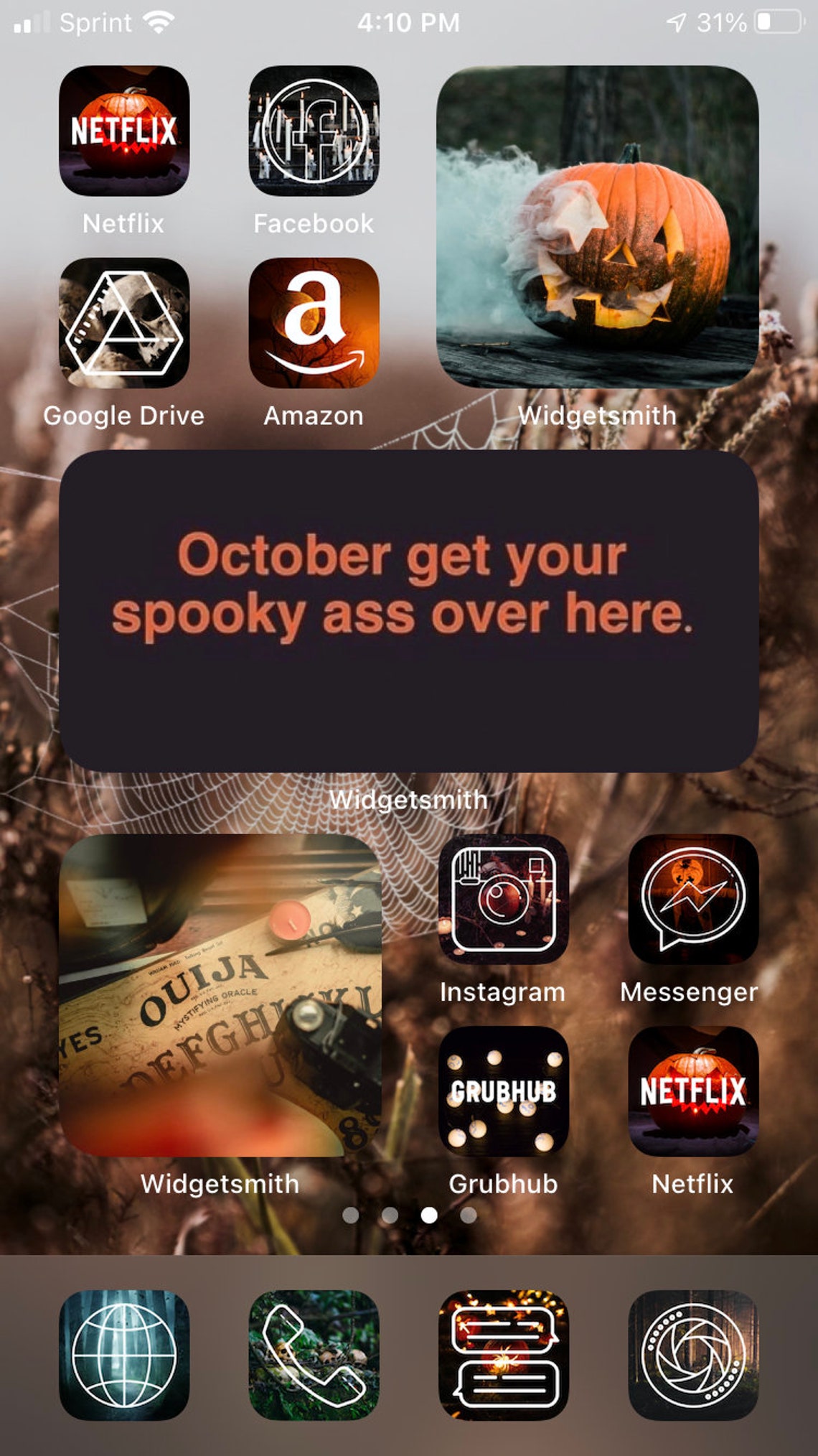A detailed screenshot of a Sprint phone's home screen is displayed. The phone shows a time of 10 p.m., with Airplane Mode enabled and Wi-Fi connected, indicated by two bars. The battery is at 31%. The wallpaper features an autumnal theme with dead leaves and a spider web, enhancing an October, Halloween vibe.

The home screen is adorned with various app icons:
- Top row: Netflix, Facebook, Google Drive, and Amazon.
- Second row features: Widgetsmith, Instagram, Grubhub, and another Netflix icon.
- Bottom row icons include: Messenger, Internet, Phone, Chat, and a circular camera icon.

At the top of the screen, there is a special Halloween-themed widget with a pumpkin design. The widget is set in a black box with orange lettering that reads, "October. Get your spooky ass over here."

Most of the app icons, except for one of the Grubhub icons, have been customized to have a Halloween theme, contributing to the overall festive atmosphere. Commonly used functionalities like Internet, Phone, Chat, and Camera are accessible via a gray bar at the bottom of the screen.